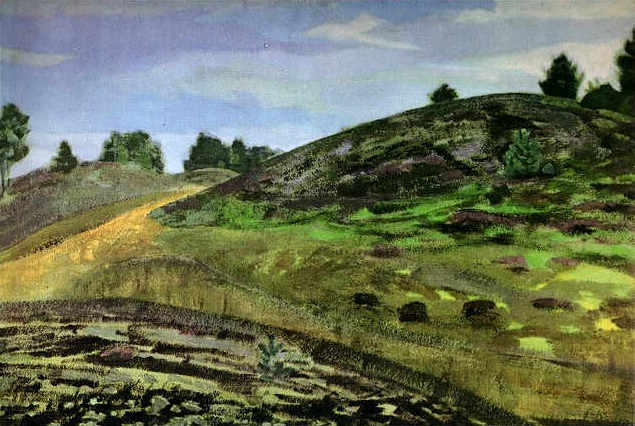The painting is a vibrant daytime landscape characterized by rolling hills and a strikingly blue sky adorned with varying shades of gray, white, and light blue clouds. Central to the image is a lush hill, its vivid green grass interspersed with patches of dark weeds and numerous gray stones. The hill features an intriguing pathway that ascends from the left-hand side toward the middle of the scene. Surrounding the hill and dotting the horizon are trees, their green leaves subtly blending into the muted backdrop. Adding to the dynamic feel are small saplings, one prominently placed at the bottom left and another on the right side of the hill. The use of bold, almost neon greens gives the grass an almost otherworldly glow, contrasting sharply with the naturalistic hues of the sky and trees. Overall, the painting employs a mix of watercolor or oil techniques to depict a richly detailed, somewhat surreal landscape.